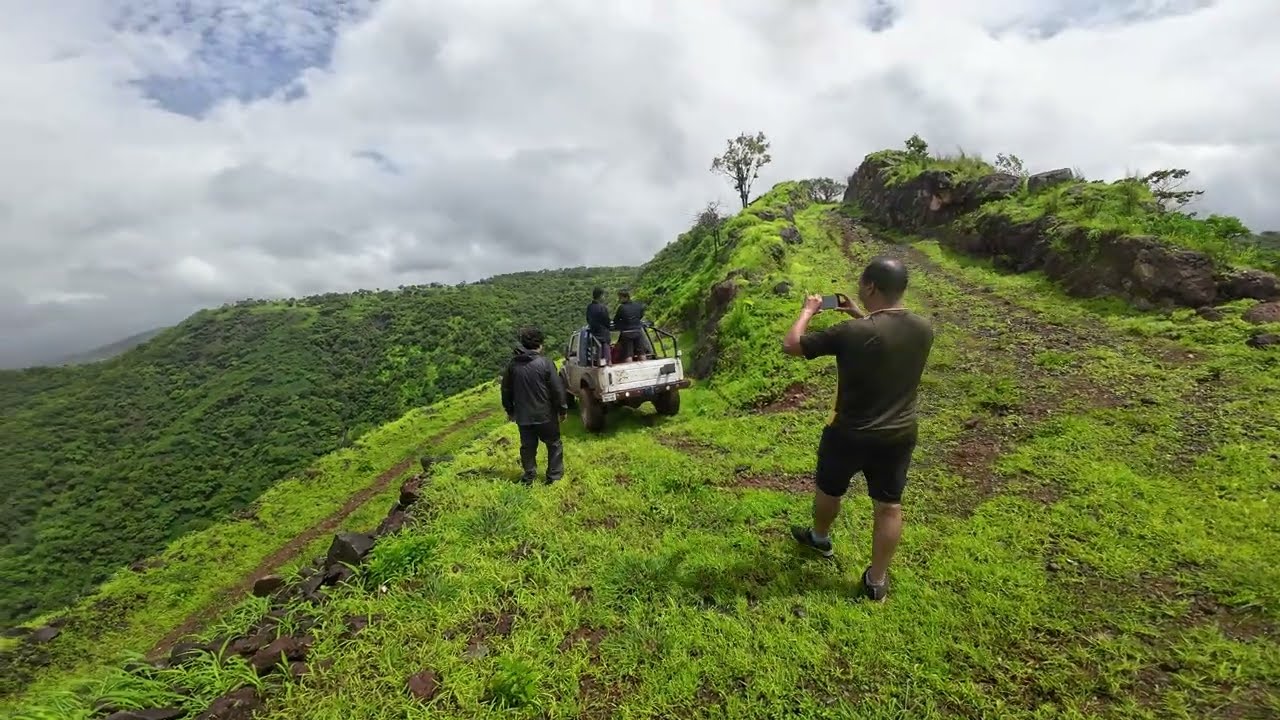The image captures an outdoor scene, likely on a lush, grassy hillside or mountain during mid-day under a bright blue sky streaked with white clouds. At the center, a white Jeep is driving up the steep terrain with two men standing in its back. Both are wearing dark attire, including hoodies and shorts. Additionally, one person wearing black pants and a black coat stands outside the Jeep on the left side. Nearby, another individual with a bald spot, dressed in a dark shirt and shorts, is using his smartphone to take a picture of the scene. The setting appears to be an adventurous hike or exploration, with a mixture of green, brown, and various shades of blue and white coloring the landscape devoid of any text or numbers. The overall aura suggests that the participants are high off the ground, possibly amidst the scenic hills of Hawaii, enjoying a shared outdoor experience.